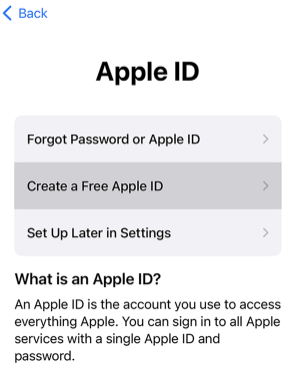The screenshot image from an Apple iPhone features a primarily white background. In the upper left corner, a blue "Back" arrow is displayed along with the word "Back." Below this, a bold black section holds the label "Apple ID." Further down, there is a light gray and dark gray tab section containing three main options:

1. "Forgot password or Apple ID" with a right-facing arrow to navigate to another screen.
2. "Create a free Apple ID" also accompanied by a navigation arrow.
3. "Set up later in Settings," again with a navigation arrow on the right.

Underneath these tabs, there is a question "What is an Apple ID?" followed by an explanatory text: "An Apple ID is the account you use to access everything Apple. You can sign in to all Apple services with a single Apple ID and password." This clear and detailed description helps users navigate their Apple ID setup options.